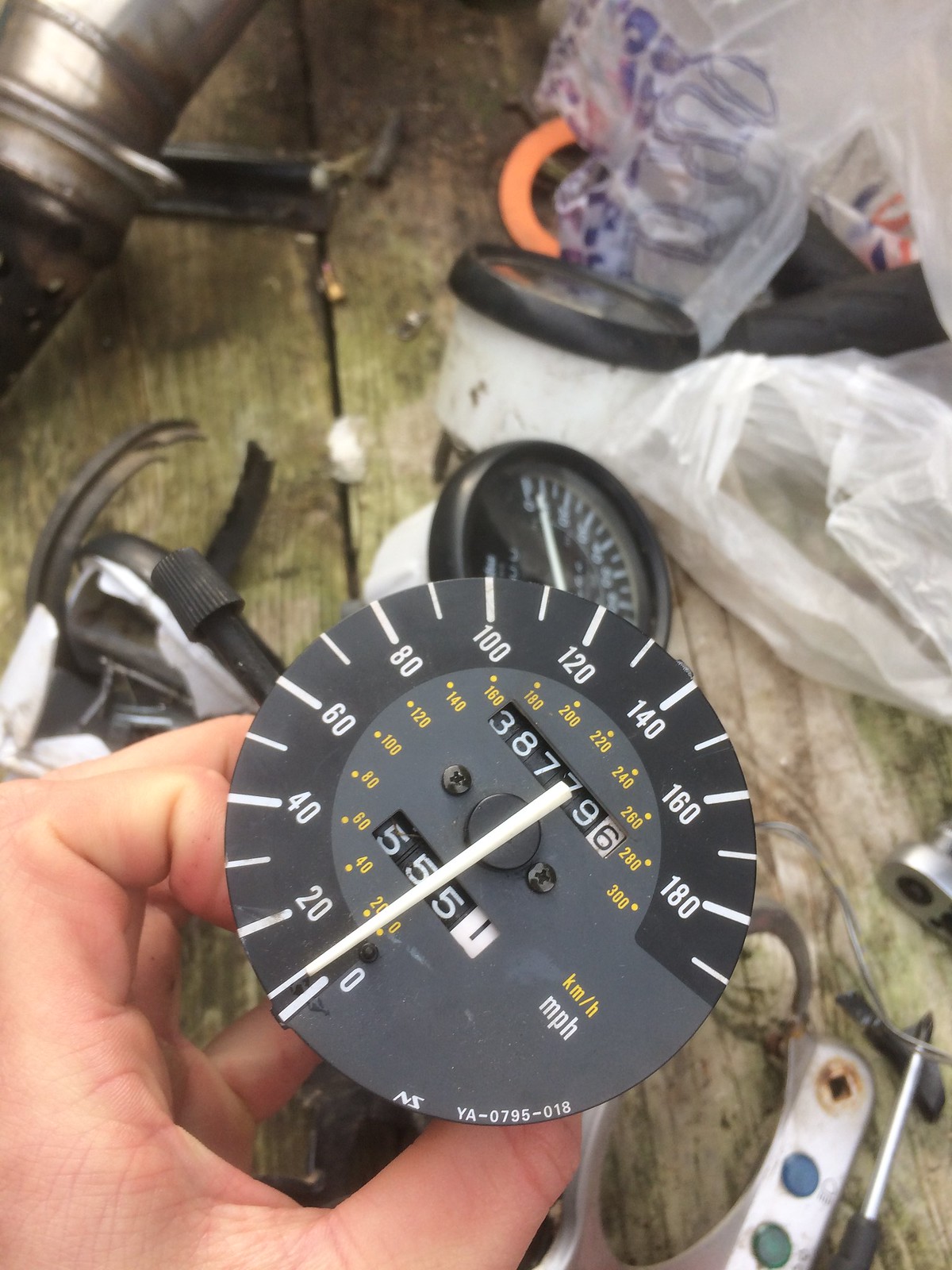A detailed photograph captures a person's left hand holding a vintage circular speedometer, prominently displayed face-up to the camera. The speedometer, with a grey background and black numbers, is marked in 20 mph intervals from 0 to 190 mph. A central needle points to zero. Concentric to the mph markings are inner markings for kilometers per hour. At the bottom edge of the speedometer, there's an inscription reading "NS YA-0795-018." Above the center, a six-digit rotary counter, currently displaying "387796," is visible, while a smaller secondary counter below shows "5551." The background reveals a cluttered workbench with various car parts, possibly including other speedometers, tools, and plastic bags, set against two slightly stained and possibly mossy wooden planks.